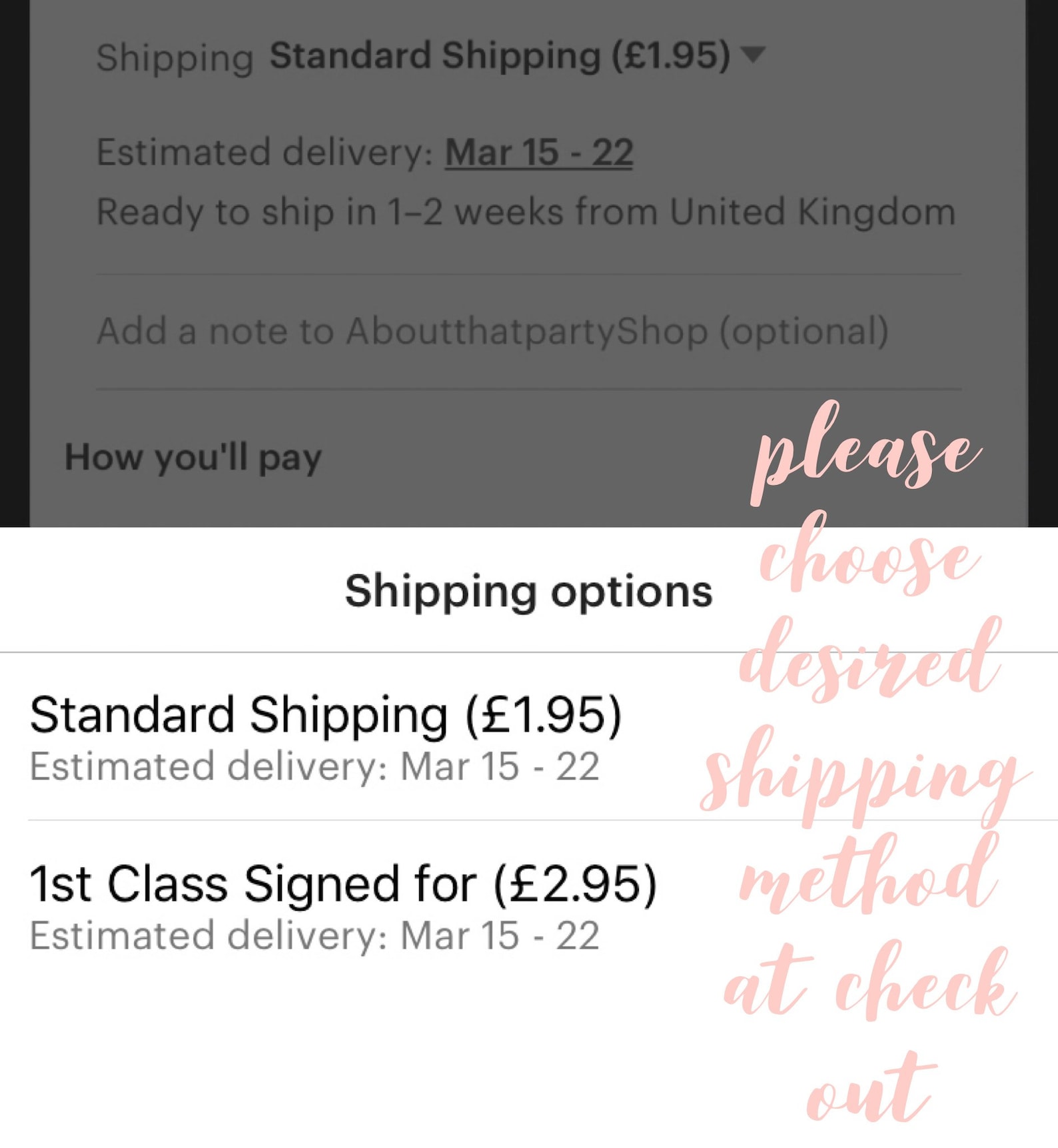This image features a meticulously organized layout showcasing shipping options. At the top, there is a cropped screenshot with a semi-transparent black filter, primarily highlighting shipping choices. The left corner of this screenshot is labeled "Shipping," with "Standard Shipping" in bold font beside a drop-down box meant for selecting other shipping methods. Centered beneath this is the phrase "Estimated Delivery Dates," followed by a note indicating the items are "Ready to ship in one to two weeks from the United Kingdom." Below this segment is an area prompting users to "Add a note to About That Party Shop" (marked as optional).

The main body of the image displays a structured text overlay against a clean background. Diagonally descending the right side, written in pink, lowercase cursive font, are the instructions, "Please choose desired shipping method at checkout." Dominating the center is the bold, black text, "Shipping Options." Situated in the bottom left corner, the image lists "Standard Shipping" along with its estimated delivery date, followed by "First Class Signed Delivery" and its respective estimated delivery dates. Finally, at the very bottom left, the image addresses the payment method with the phrase "How you'll pay."